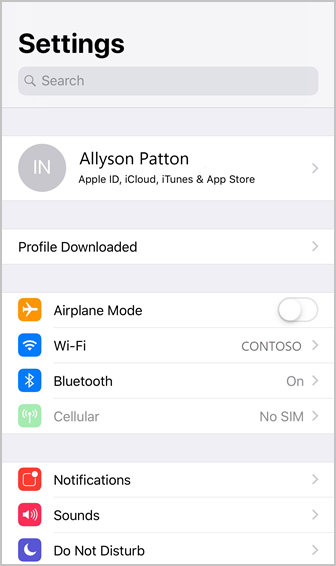In the image, Allison Patton is navigating through the Settings menu on her smartphone. The screen prominently displays the Settings title at the top, with various options listed below. The "Airplane Mode" is currently toggled to the off position, indicated by the switch aligned to the left. Allison is connected to a Wi-Fi network named "Contoso," and her Bluetooth is activated. The device does not contain a SIM card, rendering cellular services inactive.

The user interface also provides access to additional settings such as Notifications, Sounds, and Do Not Disturb. Tapping on these options, indicated by red arrows, allows deeper navigation into their respective menus. For instance, through the iCloud option under Allison's profile, she can manage her Apple ID, iCloud, iTunes, and the App Store. There's an option for downloading her profile information for easy access. 

This detailed screen captures the core functionality and customization options available within a smartphone's settings, providing insight into how users can manage their device's network connections, notifications, and personal accounts.